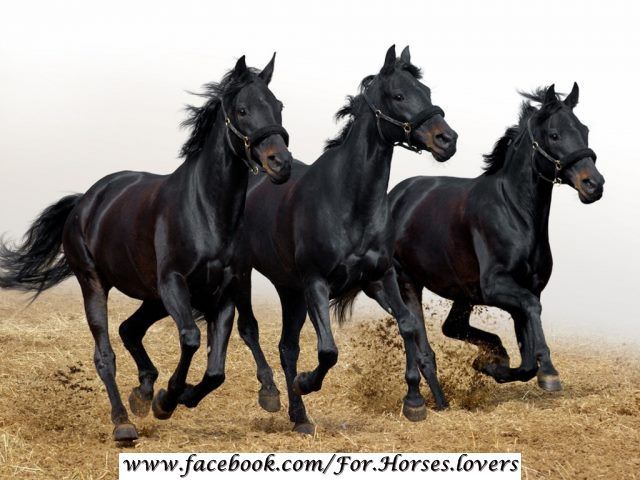The image features three stunning black stallions running side by side in unison. Their ebony bodies are highlighted with touches of brown on their faces and legs. Each horse wears a harness around its nose, though their mouths remain closed, indicating no bridles with bits. The powerful stallions appear to be galloping through a mix of dirt and hay, kicking it up in their wake, which adds dynamic motion to the scene. Their manes and tails, long and flowing, are swept back by the speed of their run. The background features a foggy, grayish-white ambiance, devoid of any detail, enhancing the focus on the horses. The entire scenery is captured from a Facebook page indicated by the link www.facebook.com/fur.horses.lovers subtly noted at the bottom.